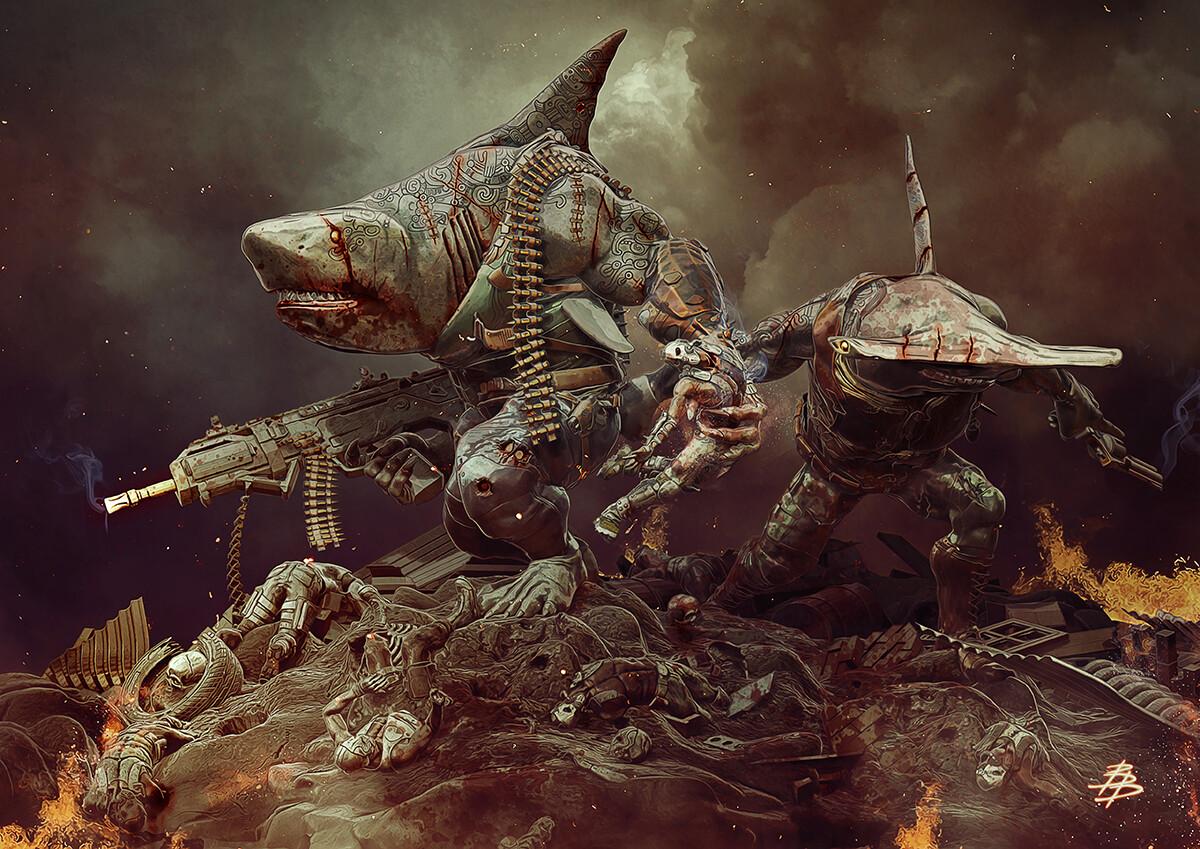The image resembles a detailed, dark-toned painting featuring two human-bodied sharks in dramatic combat attire. One character portrays a regular shark, while the other is a hammerhead shark. Both have human torsos, arms, and legs, and are outfitted in combat gear, armed with an assortment of large and small firearms, as well as knives. The regular shark has ropes of cartridges slung over its shoulder. They are depicted running through an uneven battlefield littered with skeletal remains and human corpses, significantly smaller in scale compared to the monstrous shark beings.

Their muscular bodies are marked with tattoos, and crimson blood stains are visible around their mouths, hinting at recent violence. The color palette of the artwork is somber, utilizing shades of dark and light gray, interspersed with flashes of orange, red, silver, and black. The background is dominated by a cloudy, almost black sky with sparse white clouds, enhancing the ominous atmosphere. The scene is intense and dynamic, capturing the sharks in mid-action, amidst a grim, chaotic landscape.